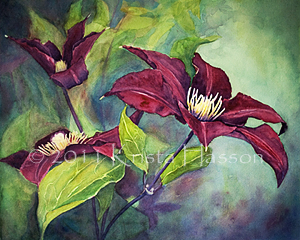This image depicts a detailed painting of a plant with three distinct burgundy flowers. The flowers have white centers where the seeds would go, and each flower is connected to the same purple stem, which features green leaves sprouting from it. The background is a mix of very blue and green watercolor-like shades, appearing blurry and giving an impression of a larger plant. There is a brighter light emanating from the top right corner, creating a contrast with the darker hues on the left side and bottom. Additionally, the painting displays a watermark that is difficult to read but seems to state "Christian Hasson, 2011." The combined elements of vivid colors and textured details enhance the beauty of this floral artwork.